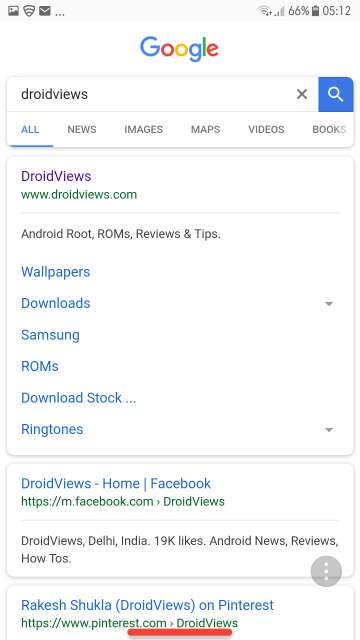The image features a Google search interface on a white background. The battery icon indicates a 66% charge, and the time is displayed as 5:12. In the search bar, the term “Joy Views” is typed, followed by a blue 'X' to clear the search. Next to the search bar, there is a blue square icon containing a white magnifying glass, symbolizing the search function.

Below the search bar, the main navigation options are underlined in blue, including options for 'All', 'News', 'Images', 'Maps', 'Videos', and 'Books'. The first search result shows the text “Joy Views” in blue, accompanied by the web address 'www.joyviews.com' in green. The description snippets include keywords such as "Android, root, ROMs," with lowercase 's' in "views". Additional links are in blue, listing "wallpapers, downloads, Samsung ROMs, download stock..."

Continuing, the image also displays dropdown arrows beside the options for 'downloads' and 'ringtones'. There’s a heading “joyviews-home” followed by a line of social media links including Facebook, Pinterest, and a green website link. The text “Rakesh Shukla (joyviews)” is in parentheses next to a Pinterest link, formatted as "https://www.pinterest.com". A right-arrow triangle icon leads to the highlighted red text under 'ST' in "Pinterest" up to 'W' in "views".